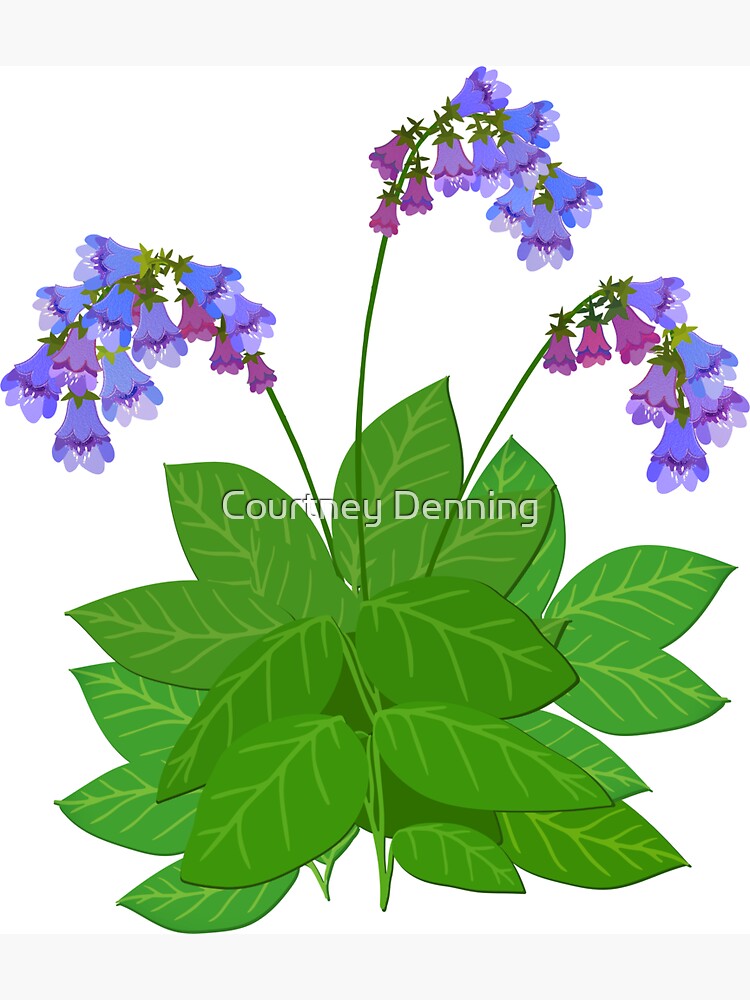This digital illustration by Courtney Denning features a pleasing portrayal of hosta plants. The artwork is set against a white background and prominently displays the artist's name as a watermark across the center. At the base, the hostas' leaves are dark green, bushy, and leaf-like with lighter veins running through them, arranged in a stacked formation. Emerging from this lush foliage are three tall, skinny green stems, each adorned with bell-like flowers in varying shades of purple and blue. Two stems lean to the right while one leans to the left, with the flowers drooping heavily downward, giving the impression of weight. The detailed, yet simplistic illustration style captures the plant's features without striving for realism, presenting a visually appealing, computer-generated image.